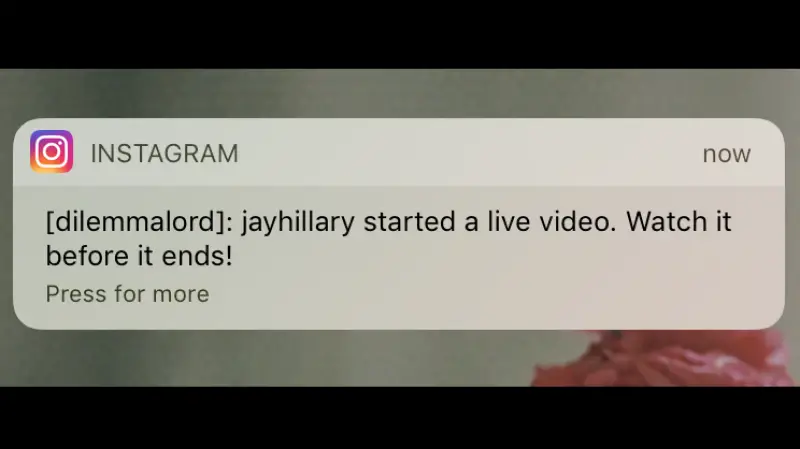This image captures an Instagram notification appearing on a user's screen, prominently displayed in the center. The notification indicates that "dilemmalord.jhillary" has started a live video, urging the viewer to "Watch it before it ends." Below this message, there is a clickable link that reads, "Press for more," inviting further interaction with the live stream. The visual composition features distinct black bars at both the top and bottom of the image, framing the notification. Behind the alert, towards the bottom right corner, a blurred background image displays what appears to be a pink flower, adding a subtle touch of color. The black bars and the background image suggest that the notification might be overlaid on a larger display, possibly a desktop or a large mobile device.